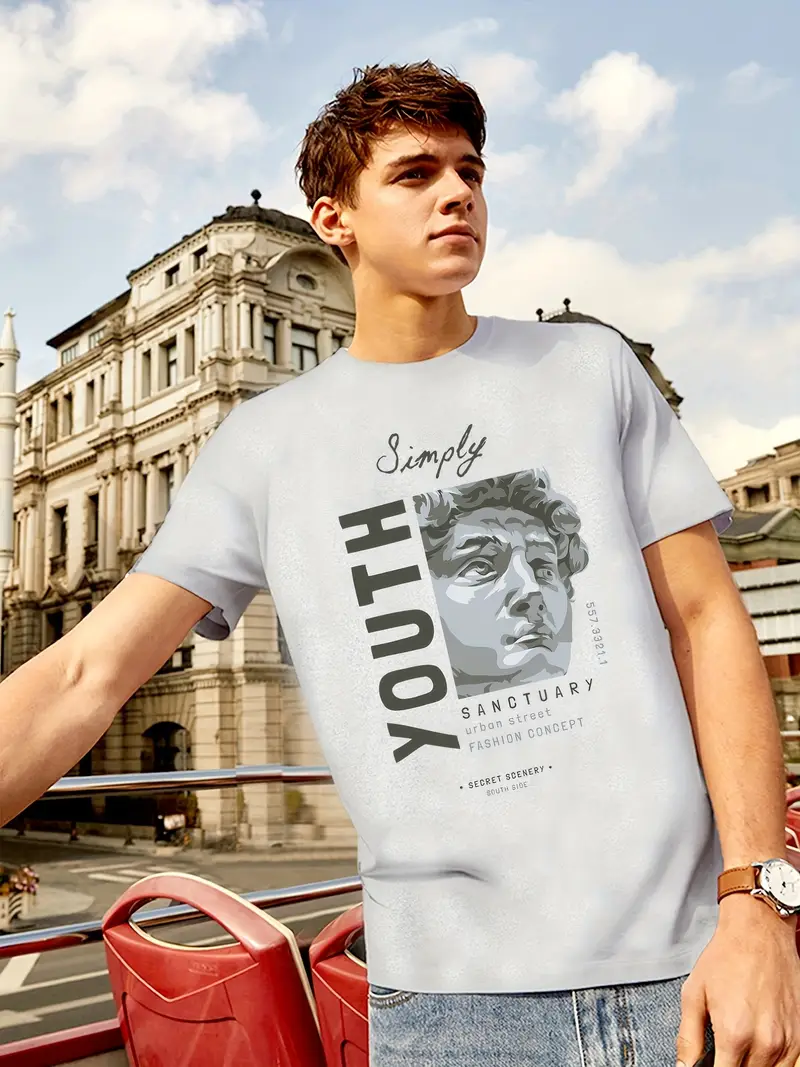A young man, identifiable by his casual attire and wristwatch, stands confidently on the upper deck of an open-top double-decker bus. The red seats behind him contrast sharply with his simple grey t-shirt, which reads "Youth Sanctuary Urban Street Fashion Concept." He is poised against the metal railing, offering a vantage point of a historic European city backdrop. The architectural marvel behind him, constructed of white brick and marble with a black roof, highlights the old-world charm characteristic of the region. His brown hair and fair complexion add to the youthful vibrance of this urban scene.